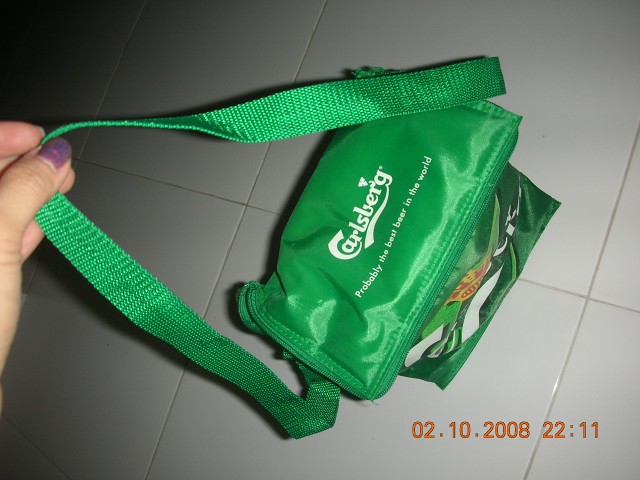The image depicts a bright green, insulated lunch bag on a white tile floor. The bag features the text "Carlsberg probably the best beer in the world" on the top, partially obscuring additional logos and colors on the front. A Caucasian hand with purple nail polish on the thumb is holding the handle, positioned in the middle left of the image. There's a noticeable light source in front, illuminating the white tile and creating a distinct shadow of the bag behind it, with the floor darkening to black in the upper left corner. The bottom right corner of the image displays the date "2-10-2008" and the time "22:11" (10:11 PM).